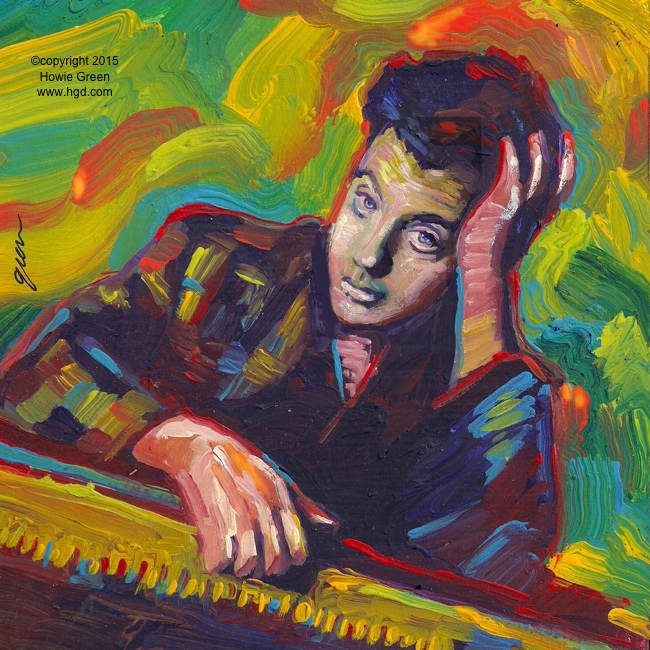The painting is an oil artwork that captures the likeness of a man resembling a young Billy Joel. Styled as a fusion between Impressionism and Picasso's techniques, it features the man with dark hair and blue eyes. He's seated and facing directly ahead, with his left hand supporting his head and his right hand on a surface resembling piano keys, though these are colored yellow. His attire is a vibrant, patchwork-like suit that integrates bright swirls of color—orange, green, yellow, red, and blue—mirroring the energetic backdrop. His skin tones blend into this palette with hues of light yellow, green, and reddish peach. Defined brush strokes emphasize the painterly nature of the work. In the top left corner, the painting is signed in black with the text: "Copyright 2015, Howie Green, www.hgd.com," and a signature is also visible on the left side.